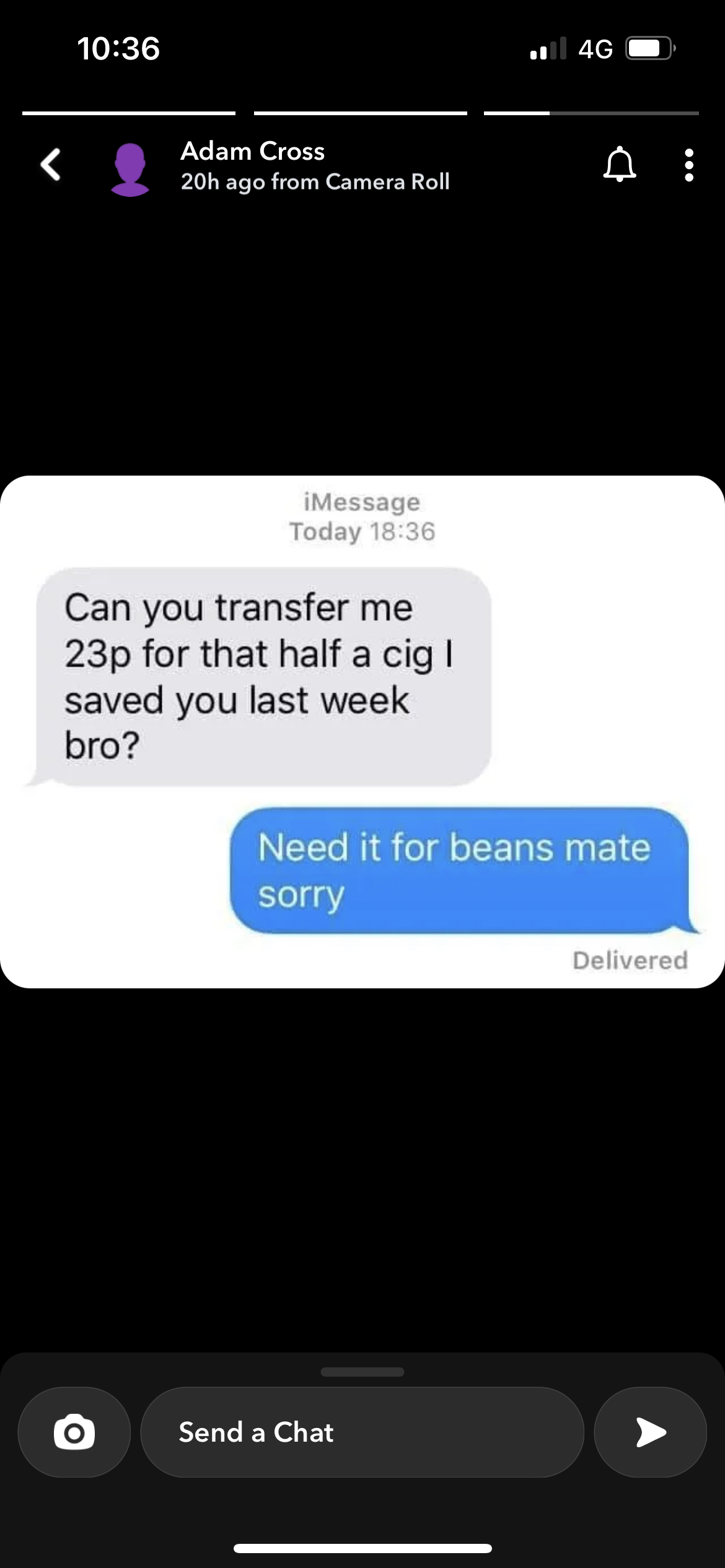This image is a color screenshot from a Snapchat, capturing a message exchange on an Android device. The overall background of the image is black. At the top, the white time display reads 10:36, and the cell and battery status icons are on the right. To the right of the username "Adam Cross," there is a white bell icon, and a left-facing arrow is on the far left. The text "20H ago from Camera Roll" appears beneath the username. 

The central part of the image is a screenshot of an iMessage conversation. The first message, in a gray bubble with black text towards the left, reads: "Can you transfer me 23p for that half a cig I saved you last week, bro?" Below it and to the right, in a blue bubble with light green text, is the reply: "Need it for beans, mate. Sorry." Underneath this is the gray text "delivered."

At the bottom of the screen, there is an input field for composing a message flanked by a photo button on the left and a send button on the right. The interface is predominantly dark, fitting the overall aesthetic of a dark user interface.